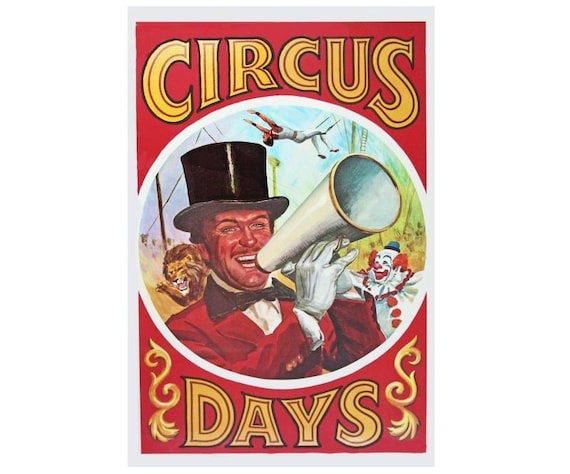This vintage poster for "Circus Days" features a vibrant red background bordered in white, with the title prominently displayed in whimsical, large yellow letters. The word "Circus" stretches across the top, and "Days" is centered at the bottom, framed by two ornate golden scrolls. Dominating the center is a large circular image bordered in white, showcasing a lively circus scene. At the heart of this illustration stands a ringmaster, exuding charisma in his black top hat, red jacket, black bow tie, and white gloves. He holds a megaphone, appearing to shout commands energetically. Surrounding him is a lively depiction of circus life: to the right, a clown in a white and red outfit with a blue cap; to the left, the fierce face of a tiger; and overhead, an acrobat performing mid-air. The entire composition captures the nostalgic excitement and lively atmosphere of a circus, drawing viewers into the fun-filled spectacle.